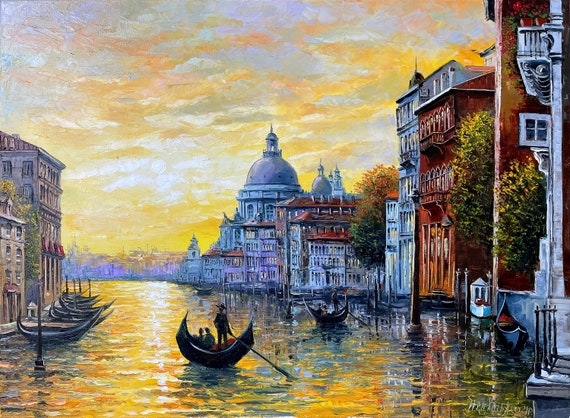This detailed oil painting captures a picturesque and romantic scene of Venice, Italy, during what appears to be the evening with the setting sun casting a golden hue across the city. In the bottom portion, a gondola is navigated by a gondolier with two passengers, setting a tranquil and traditional mood. To the left, several tethered gondolas float beside a dark brick building, while on the right, the grand palazzo and additional gondolas add to the atmospheric charm. The cityscape extends far into the background, enhancing the depth and dreaminess of the scene. The buildings, varying from dark brick to lighter shades, exhibit ornamental beauty and traditional architecture, some even featuring a hint of purple. The sky is a blend of yellow, light blue, and even light purple hues, reflecting vividly in the water, which appears yellow and white. The overall tone is a beautiful play of light and color, giving the painting an ethereal and timeless quality. Although the signature in the bottom right-hand corner is illegible, the painting's striking depiction of Venice’s canal, adorned with gondolas, intricate buildings, and the soft glow of the sunset, makes it a mesmerizing piece of art.